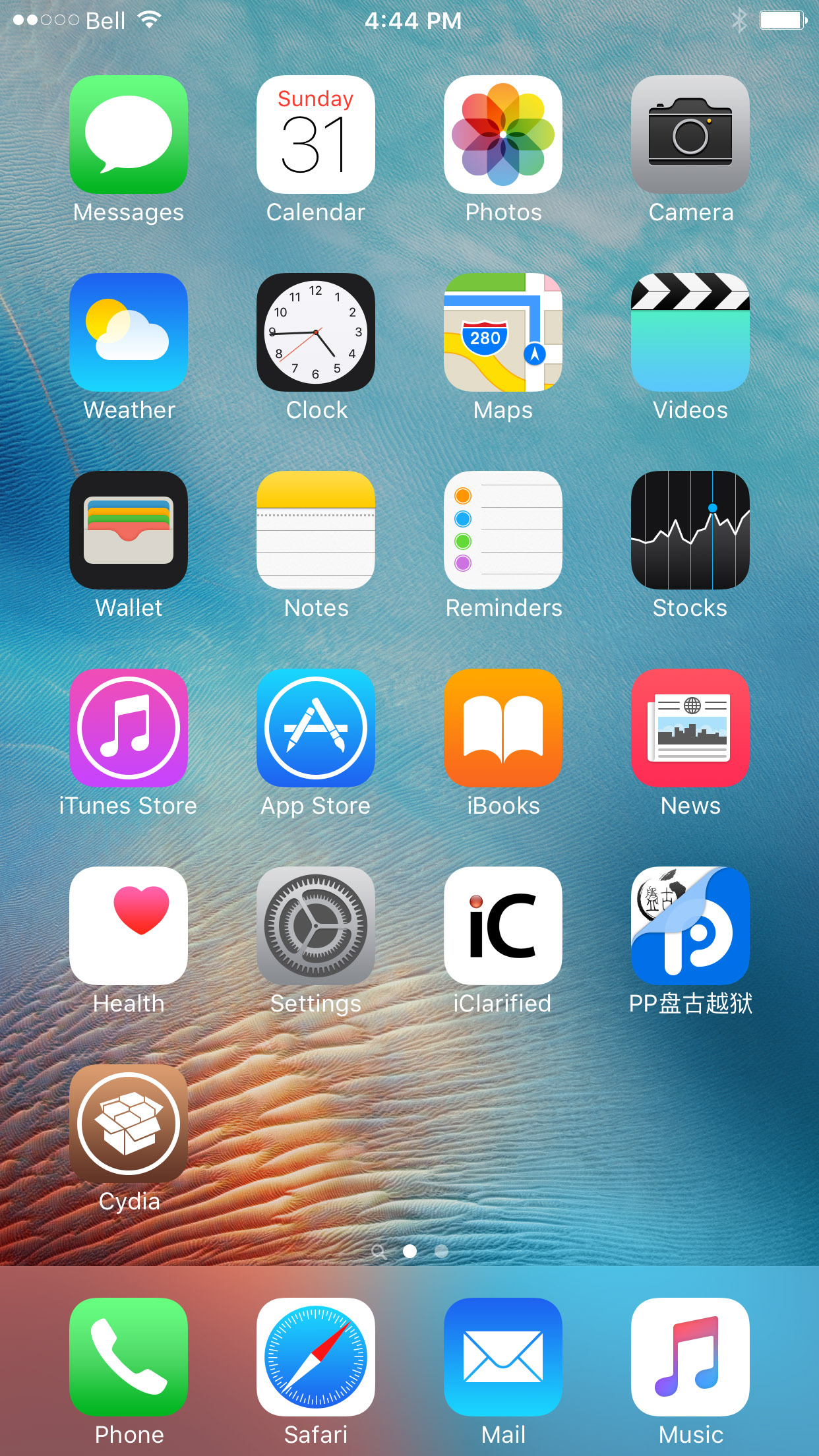The image is a screen capture of a smartphone home screen with the service provider Bell. It is 4:44 p.m., and the battery is fully charged. At the bottom, the dock features four essential applications: Phone, Safari, Mail, and Music. Above the dock, the main screen contains a variety of app shortcuts, including Messages, Calendar, Photos, Camera, Weather, Clock, Maps, Videos, Wallet, Notes, Reminders, Stocks, iTunes Store, App Store, iBooks, News, Health, Settings, iClarified, an unidentified Taiwanese or Chinese app, and Cydia. The background wallpaper is an abstract smear featuring a multitude of colors.